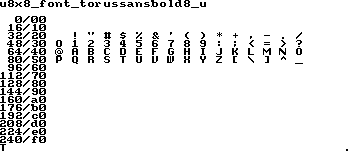The image showcases a white background with bold black text, consisting exclusively of characters and numbers. At the top, it denotes "U8X8_font_torus-sans_bold_8_u," succeeded by a structured series of alphanumeric strings and corresponding decimal values. The sequence is as follows:

- 0 / 0
- 00 / 16
- 10 / 32
- 20 / 48
- 30 / 64
- 40 / 80
- 50 / 96
- 60 / 112
- 70 / 128
- 80 / 144
- 90 / 160
- a0 / 176
- b0 / 192
- c0 / 208
- d0 / 224
- e0 / 240
- f0

Further down, a variety of symbols and characters are displayed, including the entire range from 'a' through 'z' and numbers, evocative of a miniature keyboard layout.

A single, small black dot is noticeable to one side. The overall image quality is excellent, with the font being exceptionally clear and legible, free from any pixelation or blurring. There are no additional images or elements present aside from those described.

---